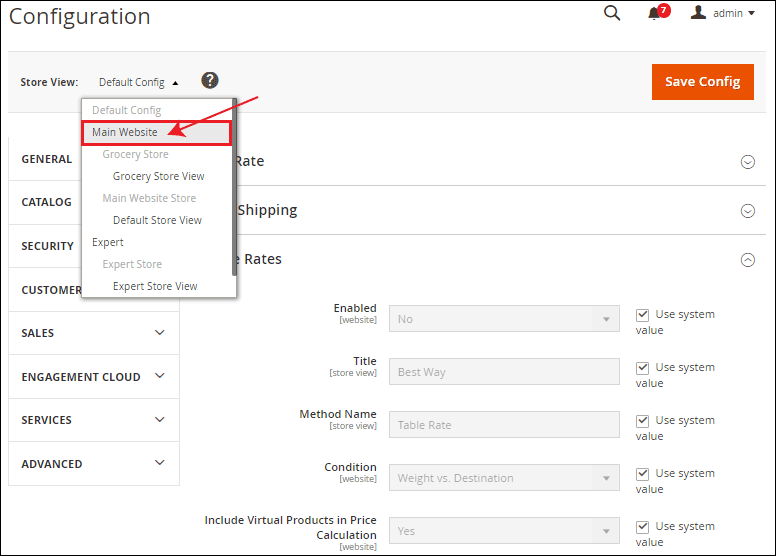This image showcases a detailed screenshot of a configuration interface. In the upper left corner, the heading "Configuration" is prominently displayed. On the upper right corner, a search icon is visible adjacent to a notification bell indicating seven new alerts, and a profile icon labeled "Admin."

Directly below, a section titled "Store View" is visible with a dropdown menu. This menu is expanded to reveal options, and the option "Main Website" is highlighted with a red rectangle and a red arrow pointing to it. To the right of this dropdown, a noticeable orange button labeled "Save Config" is displayed.

The left-hand sidebar lists various options such as "General," "Catalog," and "Security." Text in the central part of the screen, partially obscured by the dropdown, includes words like "rate," "shipping," and "rates."

Continuing down the left sidebar, additional options are named, including "Customer," "Sales," "Engagement," "Cloud," "Services," and "Advanced." Towards the bottom right of the interface, there are several fields and dropdown boxes labeled "Enabled Website," "Title," "Store View," "Method," "Name," "Condition," "Website," with two final dropdown options pertaining to "Virtual Products" and "Price Calculation."